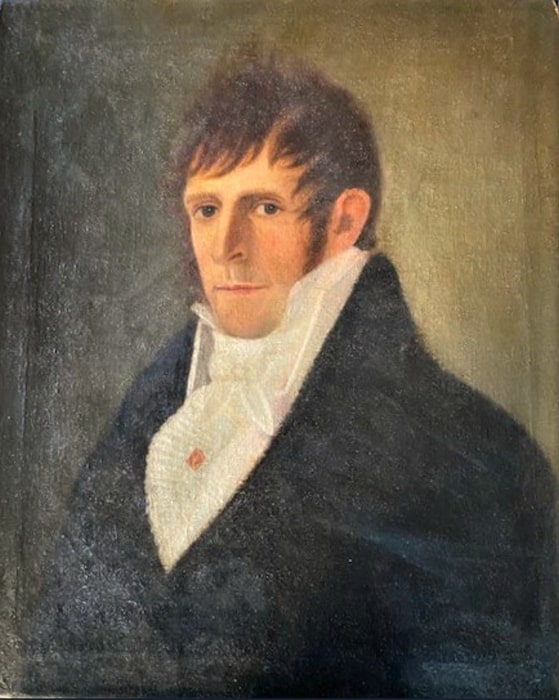The image is a vertical rectangle scan or photograph of an old, weathered oil painting, likely from the 1700s or 1800s. The background is a mix of light and dark shades of brown and green, fading more prominently on the left side. The painting features a fair-skinned man in the center, viewed from the chest up, staring directly at the viewer with dark eyes. He has brown hair combed forward in an unkempt, emo style popular during the Napoleonic Wars, with long sideburns and ears fully exposed. His face is expressionless, with a straight, somewhat narrow nose and a straight-lipped, stern demeanor. The man wears a formal, dark blue or black coat over a high-collared white shirt, which puffs out into frills at his chest. A notable detail on his attire is a gold brooch or button on the ruffled part of his shirt. The painting exudes an air of historical significance and aristocratic elegance, akin to portraits from the novels of Jane Austen.